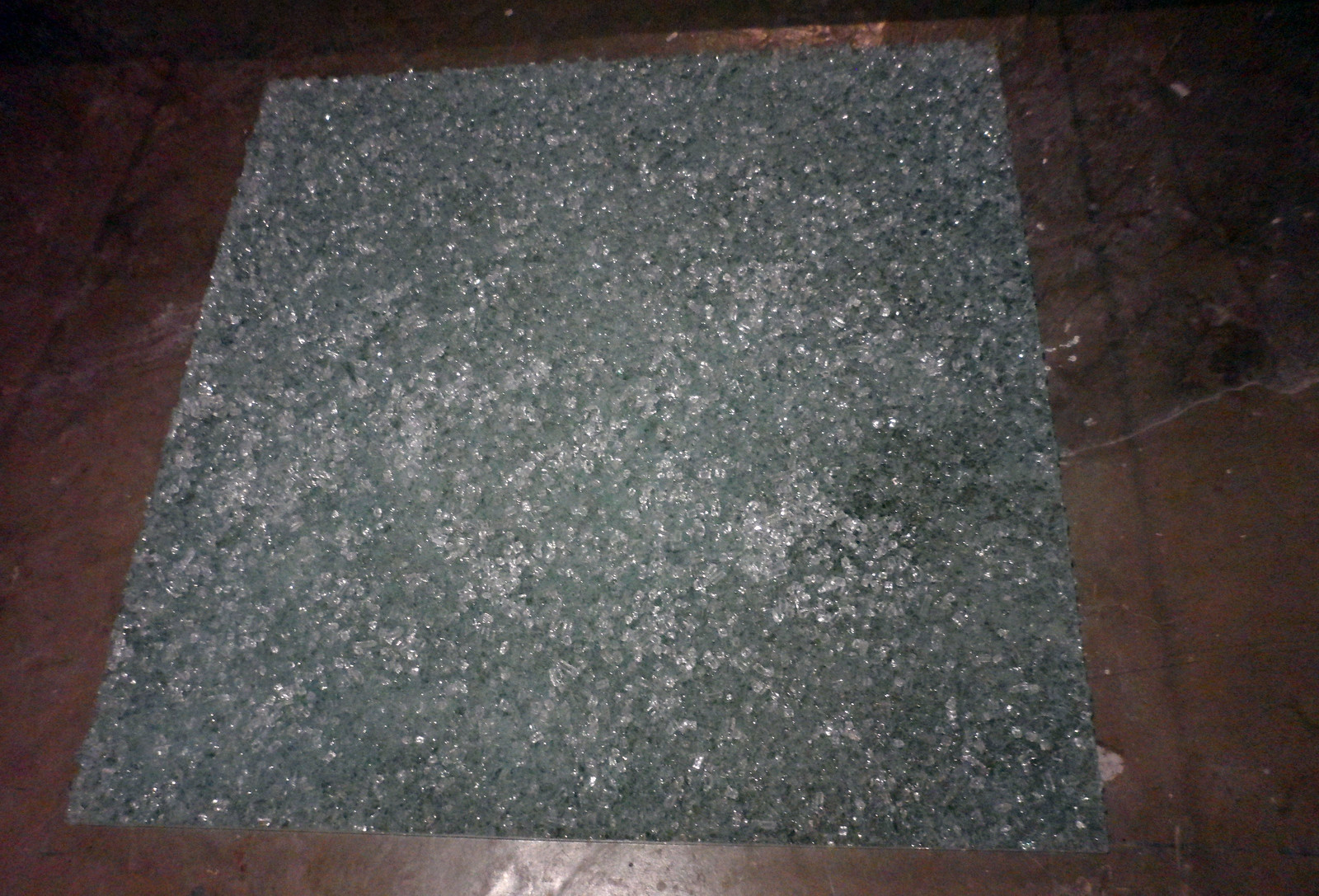The image is a photograph of a gray rectangular object with various shades of gray, including dark gray, light gray, and silver-like hues, which gives it a shimmering appearance. It may be made from fabric, tile, or paper. This object is placed on a polished brown floor, which could be tiled or wooden, and has patches or streaks of black throughout. The gray rectangle, measuring approximately 18 inches by 12 inches, is predominantly gray with splashes of white, and it slightly rises from the floor at the top end, suggesting it might be held up by something. The brown floor surrounding the gray object is visible with some reflections of light at the bottom of the image, emphasizing the polished nature of the floor.